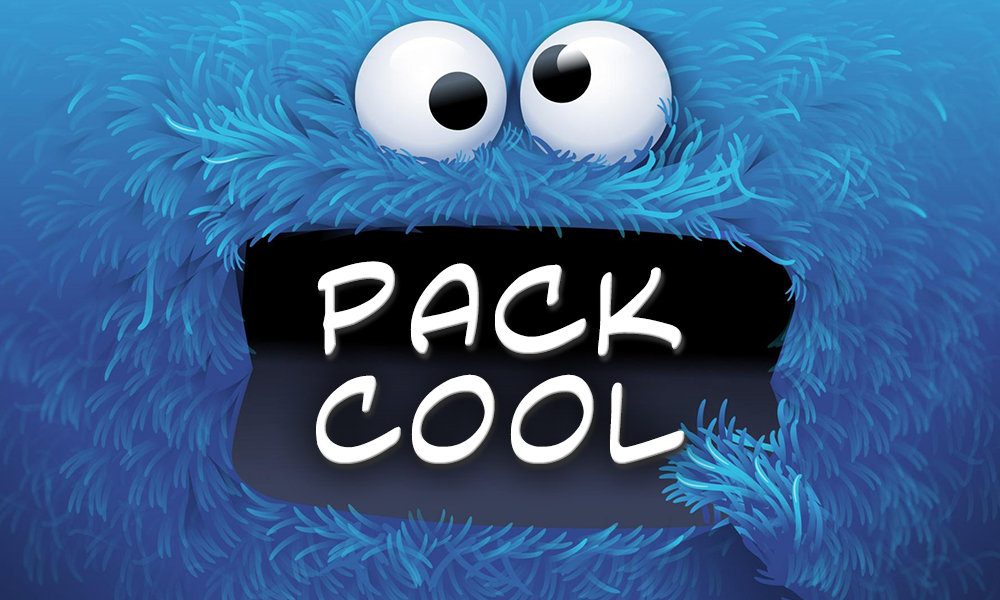The image is an advertisement featuring an illustration that closely resembles the Sesame Street character, Cookie Monster. Dominating the entire image, the character is portrayed with various shades of blue fur, giving him a fuzzy, textured appearance. His large googly eyes, consisting of white spheres with black pupils, are positioned at the top of the image and are slightly askew, with one eye looking straight ahead and the other glancing upward. Below his eyes is a wide, black, open mouth that has a distinct square shape with rounded sides, creating the impression of a hinged puppet mouth. Inside his mouth, the words "PAC COOL" are displayed in bold, white, capital letters, one word above the other. In the lower right corner of the mouth, an appendage resembling a small blue hand or paw reaches into the mouth, adding to the dynamic composition. The overall visual effect is engaging and whimsical, capturing the playful essence of Cookie Monster while clearly presenting the textual element of the advertisement.